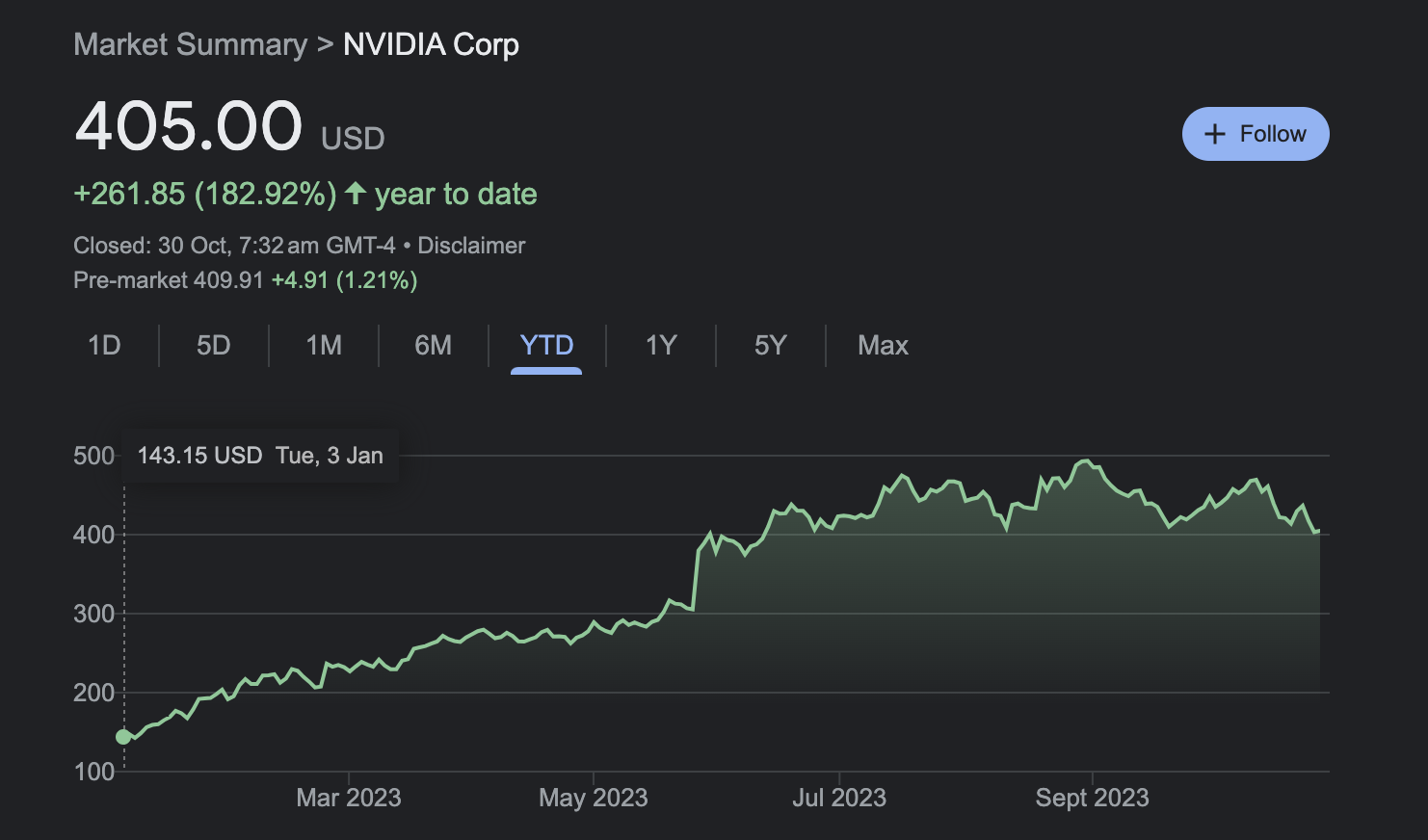The image presents a detailed Market Summary for NVIDIA Corporation. Set against a black rectangular background, the summary prominently displays several pieces of key information. In the upper left corner in gray text, it reads "Market Summary." Below, there is the white text "NVIDIA Core," followed by "405.00 USD" beneath it. Under the price, in green text, it states "+261.85," indicating an increase of 182.92% year-to-date. Adjacent to this, on the right, is a blue "Follow" button.

The details note that this summary pertains to the NVIDIA Core stock, which closed on October 30th at 7:32 a.m. GMT. At the bottom section of the image, there is a graph illustrating the stock's performance over time. The graph has options at the top to view different time ranges, labeled "1D, 5D, 1M, 6M, YTD, 1Y, 5Y, and Max," with "YTD" (year-to-date) highlighted.

The vertical axis on the left side of the graph scales from top to bottom, marked at increments of 100 from 500 to 100. The horizontal axis along the bottom shows periodic timestamps: March 2023, May 2023, July 2023, and September 2023. The graph itself features a green wiggly line that starts near the 100-mark before climbing steadily to reach around the 400-mark past September. This visual representation underscores the significant upward movement of the NVIDIA stock over the specified period.